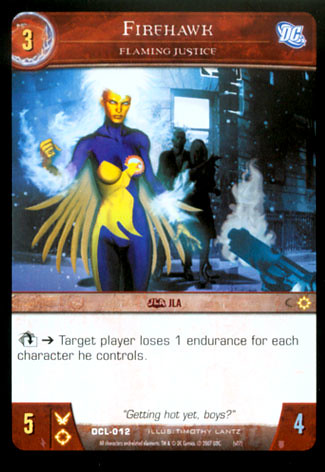The image shows a playing card from a DC Comics-themed game. The card features a striking illustration of a character named Firehawk, Flaming Justice. Firehawk appears as a woman with long blue hair that seems to be on fire, extending flames down both arms and onto her gloves. She is dressed in a distinctive blue and white suit with feathers attached to her back, giving her a winged appearance. Surrounding her are dark silhouettes of other figures, one of which points a gun at her, all against a predominantly blue background. 

The top section of the card has a rust-colored trim, with a yellow number 3 in the upper left corner, likely indicating a power or point value, and a DC Comics icon in the top right. The card's name, "Firehawk, Flaming Justice," is prominently written in white text. Below the image, there is a strip of brownish-red color, followed by text detailing the card's effect: "Target player loses one endurance for each character you control." The bottom corners of the card display a yellow number 5 on the left and a teal number 4 on the right, possibly indicating additional game metrics.